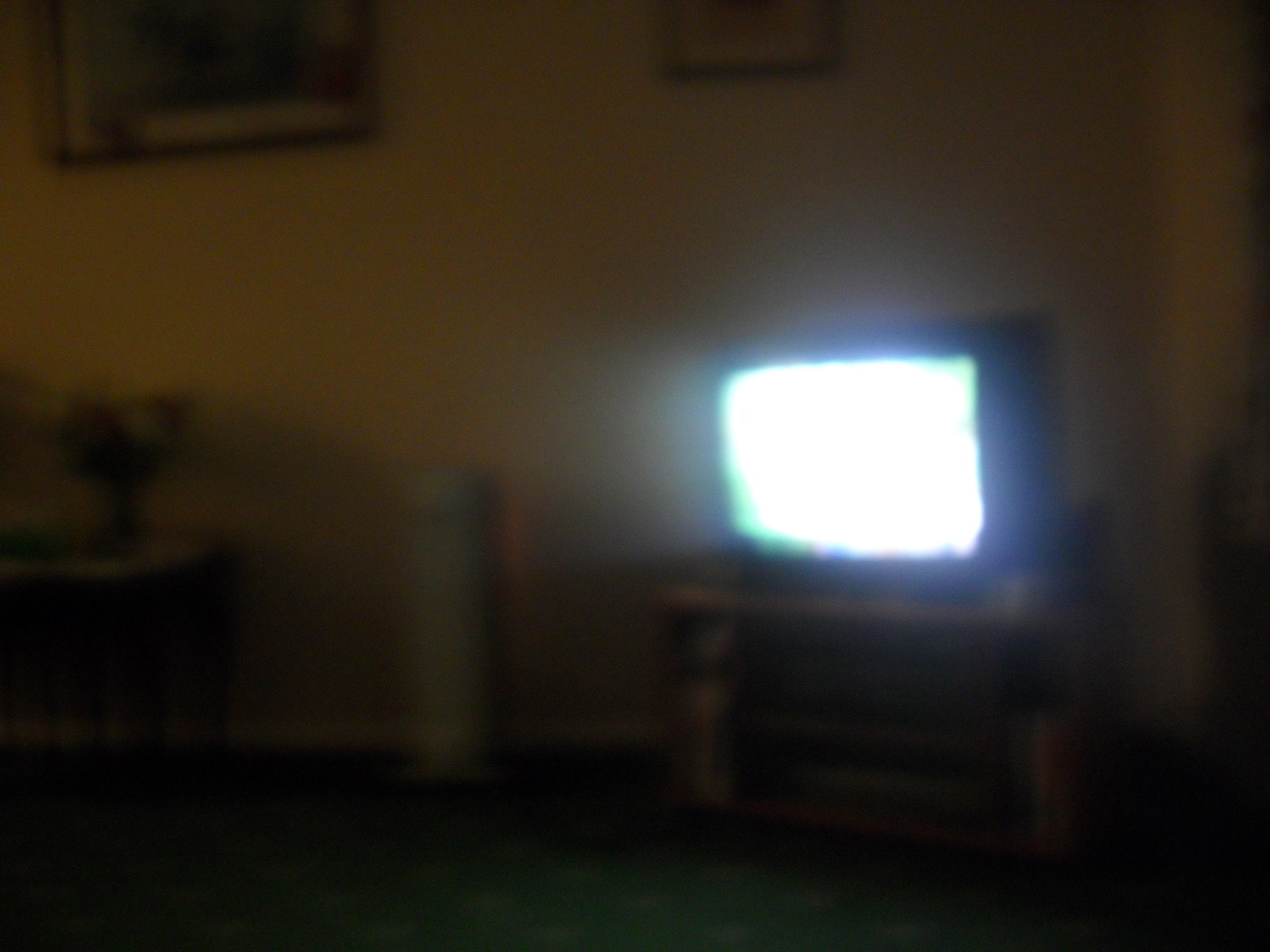This image depicts an out-of-focus scene of a dimly lit room. The focal point is an old-style television positioned towards the middle-right side, emitting a soft, white and blue-green glow from its screen, which offers no discernible details. The television, encased in an outdated, boxy frame, sits atop a lightly colored table. To the left of the television, a tall, light-colored object—potentially a fan or air purifier—stands prominently. Further to the left, there is another table adorned with a bouquet of flowers. The background showcases a light-colored wall adorned with pictures, though the specifics are obscured by the darkness.